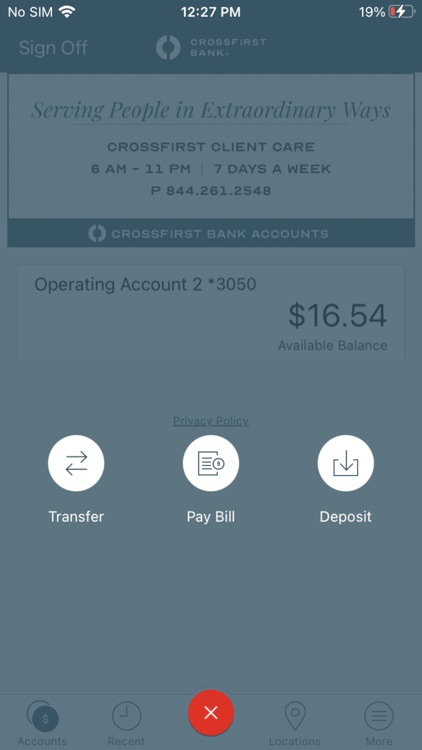**Detailed Caption:**

This image is a screenshot taken from an iPhone, displaying an app presumably belonging to Cross First Bank. In the top left corner, the screen indicates that there is "No SIM," while further to the right, the Wi-Fi symbol is visible. Centered at the top, the time is displayed as "12:27 p.m.," and on the far right, the battery indicator shows "19%" with an accompanying symbol suggesting the phone is currently charging.

Faded in the background, the app or website interface provides helpful information. At the top, it displays "Cross First Bank" alongside a logo. Below this, a motto reads "Serving people in extraordinary ways." The section lists "Cross First Client Care" with available hours from "6 a.m. to 11 p.m., seven days a week," followed by a contact phone number.

A colored banner stretches across the screen with the text "Cross First Bank Accounts." Underneath, a white rectangle shows the details of the "Operating Account" including the account number and the available balance of $16.54.

The screenshot indicates that the user has various action options, highlighted in white buttons: "Transfer," "Pay Bill," and "Deposit." Additionally, a circle with a red 'X' icon is located beneath these options, providing an easy way to exit the current screen.